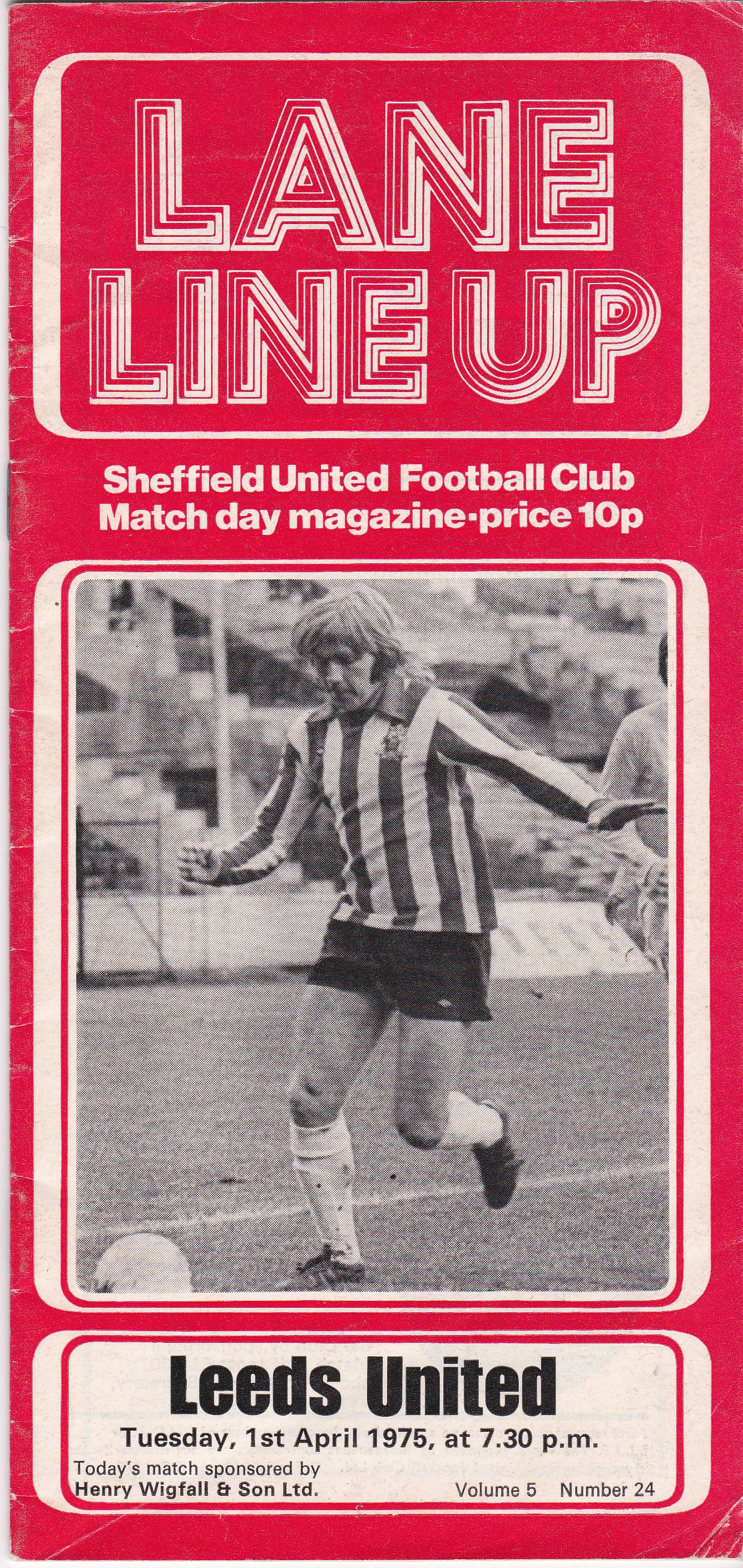This is a vintage match day program from an English soccer game between Sheffield United and Leeds United, dated Tuesday, 1st April 1975 at 7:30 PM. The program, titled “Lane Lineup,” is designed as a vertical rectangle with a red background. At the top, a white rectangle features the title “Lane Lineup” in white and red lined text. Below this, the text states “Sheffield United Football Club Match Day Magazine, Price 10p.” Dominating the center is a black-and-white photograph of a soccer player on a well-maintained field. The player, with long hair, wears a striped long-sleeve polo shirt, dark shorts, and knee-high white socks, and is captured mid-kick, dribbling a white soccer ball. The bottom of the cover highlights the match details in large black text: “Leeds United, Tuesday, 1st April 1975 at 7:30 PM.” Additional details note the match is sponsored by Henry Wigfall and Sons Limited, and it is Volume 5, Number 24.